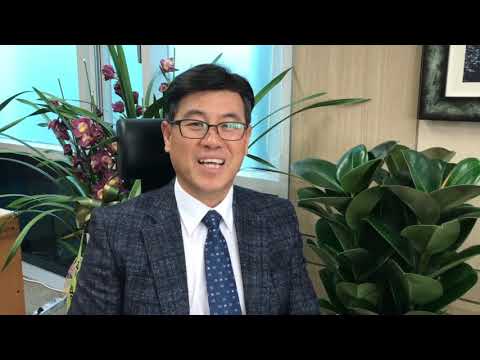In this detailed image, we see an older Asian male sitting in a black leather office chair at the center of the composition. He has black hair with some graying at the sides, and it is neatly combed to the left. He wears black-rimmed glasses, a white collared button-up shirt, a blue tie adorned with small white spots, and a dark blue tweed suit jacket. His friendly smile is directed towards the camera.

The setting appears to be an office environment in the middle of the day, framed by letterbox bars at the top and bottom of the image, suggesting it might be a still from a video. Behind him, a wood-paneled wall can be seen, adorned with a framed picture in a green frame positioned in the top right corner. To his right (bottom left corner of the photo), a potted plant with thick, glossy green leaves adds a touch of nature to the scene. Directly behind him, there's another plant with long, slim leaves and purple flowers, which adds more color and a lively ambiance to the space. Additional windows are visible in the top left corner, providing natural light that enhances the overall brightness of the room. The colors in the image include varying shades of brown, dark gray, blue, white, tan, green, and light blue, contributing to a warm and professional atmosphere.